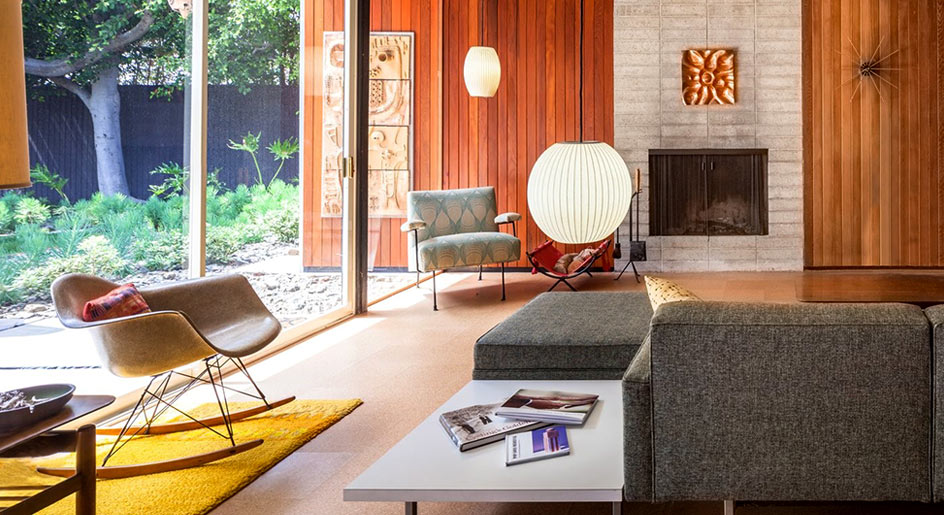This photograph captures a captivating mid-century modern living room characterized by its warm color palette and thoughtful design elements. The left side of the room is dominated by large, floor-to-ceiling glass sliding doors that overlook a serene backyard filled with tall trees and abundant greenery. Directly in front of these windows lies a light grey rocking chair positioned on a vibrant yellow rug. 

The fireplace, located towards the right side, is constructed from white, symmetrical bricks and features a striking golden sculpture above it. Additionally, the fireplace area includes a set of fireplace tools, such as a poker and a small shovel. Hanging from the ceiling are modern, round lantern-style lights that add a soft, ambient glow to the space.

Adjacent to the fireplace is a sleek, dark grey couch accompanied by a matching ottoman and a nearby white coffee table topped with magazines. The room also features a blue chair and another small wooden side table, which holds an ashtray with cigarette butts. 

A standout element of the room is the wood paneling on the walls, displaying two distinct shades: a deep, rusty red and a warm orange. The red panels continue seamlessly into the exterior design of the house. Additionally, a striking mid-century sunburst clock with spiky radial points adorns one section of the wall, matching the warm tones of the wood paneling. Overall, the room blends warm hues, modern furniture, and classic mid-century details to create a harmonious and inviting space.